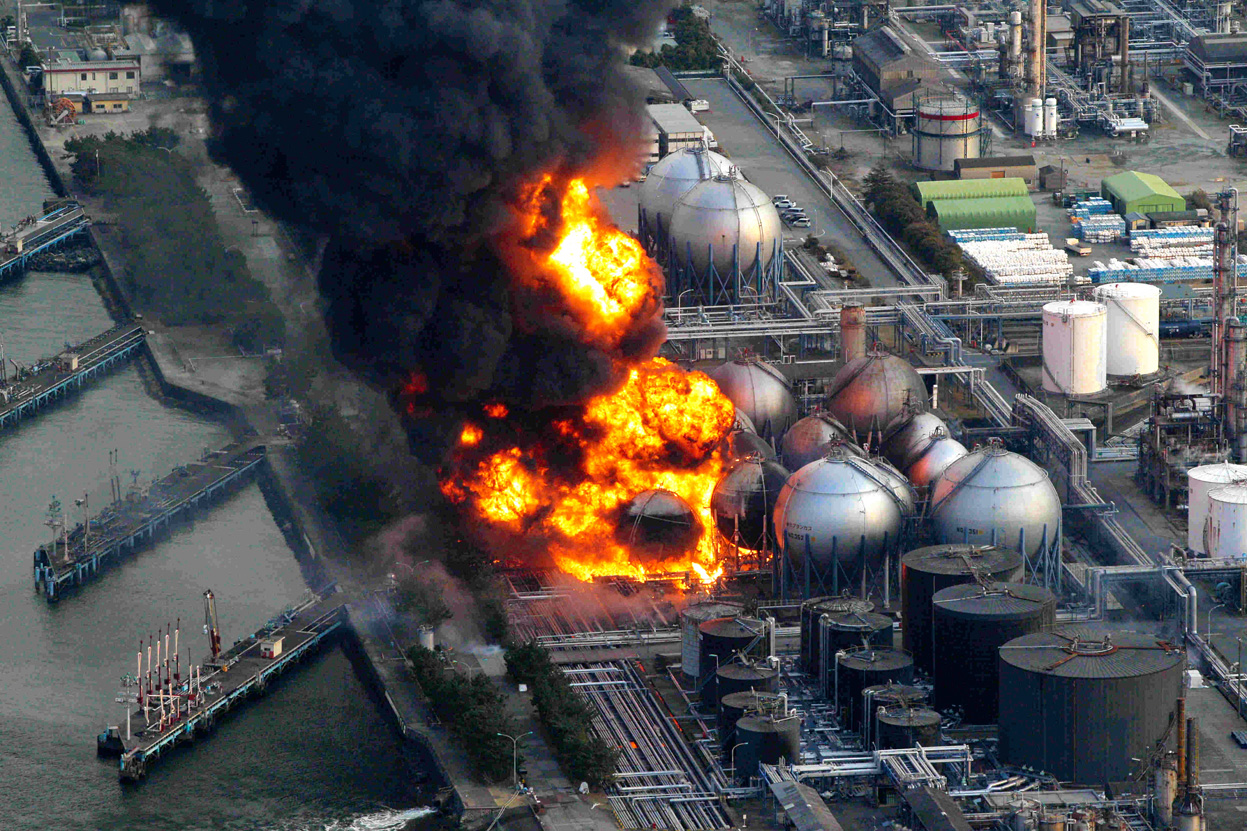This aerial photograph captures a large, intensely bright orange-yellow fire with thick black smoke billowing skyward in the center of an oil refinery or industrial facility. The sprawling complex is situated by a body of water, most likely the ocean, visible on the left side of the image where four docks stretch diagonally from the shoreline. A border of trees separates the water from the industrial area. The refinery itself consists of an array of structures, including large metallic tanks, some spherical and others oval-shaped, supported by beams. Additional infrastructure like tubes, pipes, and small garage-like buildings spread across the scene. An empty parking lot and cars can be seen, and there are no ships docked or people visible, nor are there any firefighters on the scene. This dramatic view is likely captured from a drone, helicopter, or aircraft.